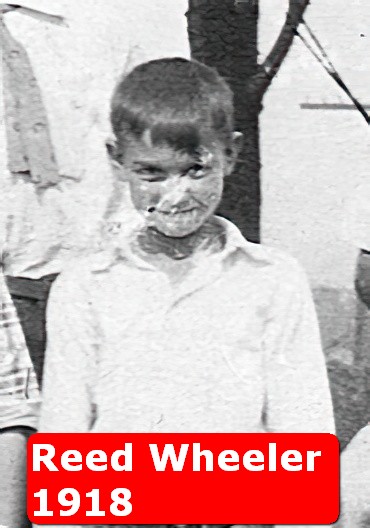This is a black-and-white photograph from 1918 featuring a young, smiling boy named Reed Wheeler, possibly around ten years old. Reed, who sports short hair with bangs falling over his forehead, is at the center of the image, tilting his head down slightly, and wearing a white shirt. To his left and right, though mostly cut off, are two adults. One figure behind him is distinguished by an elbow and a torso clad in a white shirt with a tie, while the other is partially visible, wearing a striped shirt. The background includes a tree trunk and indistinct ground. Despite showing signs of age, with some scratches around his nose and mouth, the photograph is in relatively good condition for being over a century old. At the bottom of the photo, prominently labeled in red with white letters, is the name "Reed Wheeler 1918," indicating the identity and date.